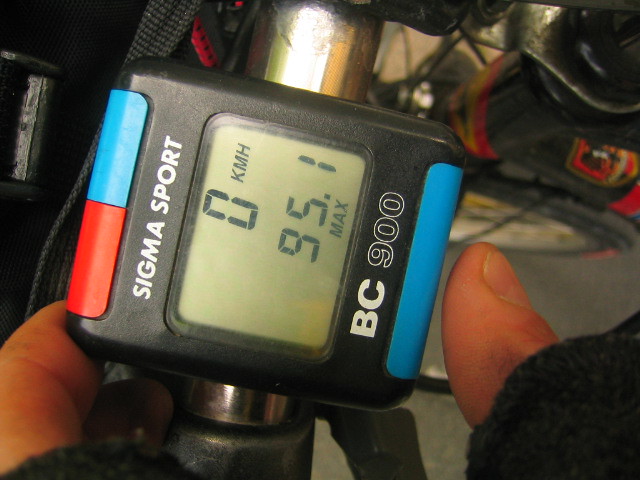This color photograph captures a close-up view of a bicycle's frame and a handlebar-mounted digital device, as seen from the perspective of the rider. The silver bike frame ascends diagonally from the center of the image. Affixed to the frame is a black device with a black casing, prominently positioned in the photograph. The device features a red button and a blue button at its top, and an additional blue button at the bottom. Just visible at the edges of the black device are a rider’s thumb and index finger, suggesting interaction with the gadget.

The device bears the label "Sigma S-I-G-M-A Sport" and includes an LCD screen displaying the reading "0 KMH 95.1 Max." Above the lower blue button, the model identifier "BC 900" is inscribed, with "BC" in white lettering and "900" outlined in white, filled with black. The background reveals a blurred assortment of indistinguishable items. The photograph is notably wider than it is tall, providing an immersive, detailed glimpse into the rider's perspective and equipment.